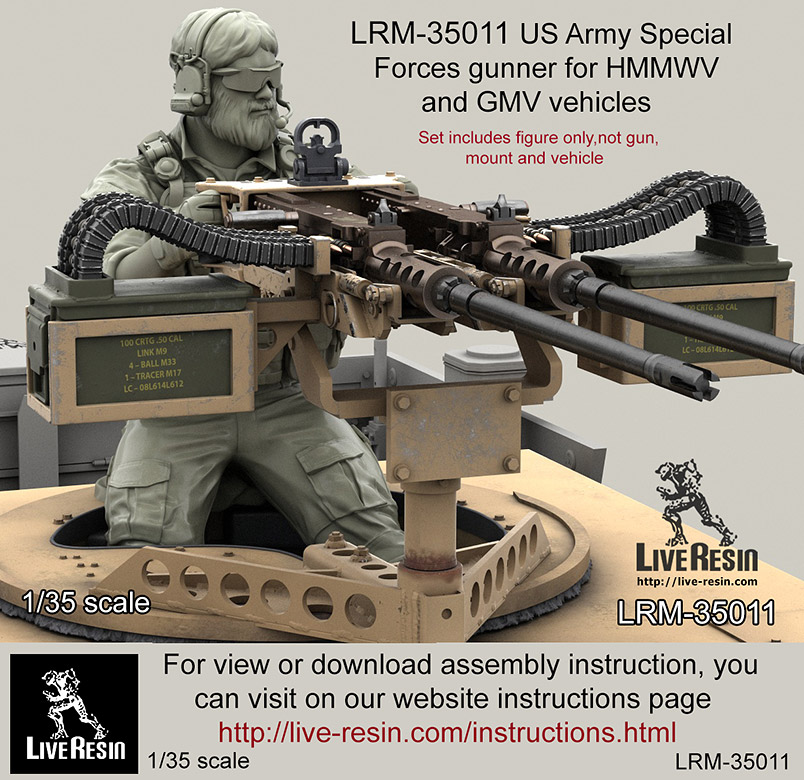The image features an advertisement for a 1:35 scale resin model kit from Live Resin, designated LRM-35011. The model portrays a U.S. Army Special Forces gunner, complete with long hair, a full beard, and goggles paired with a headset. Clad in detailed arming gear, the figure is depicted emerging from the turret hatch of a Humvee or GMV vehicle, manning a dual .50 caliber machine gun. Though the dual-barrel gun dominates the foreground, the text clarifies that the set includes only the figure, excluding the gun, mount, and vehicle components. Key details include the model name "LRM-35011 U.S. Army Special Forces Gunner for HMMWV and GMV vehicles," a reminder to visit their website for assembly instructions (http://live-resin.com), and prominently displayed branding and scale information in the corners of the advertisement.